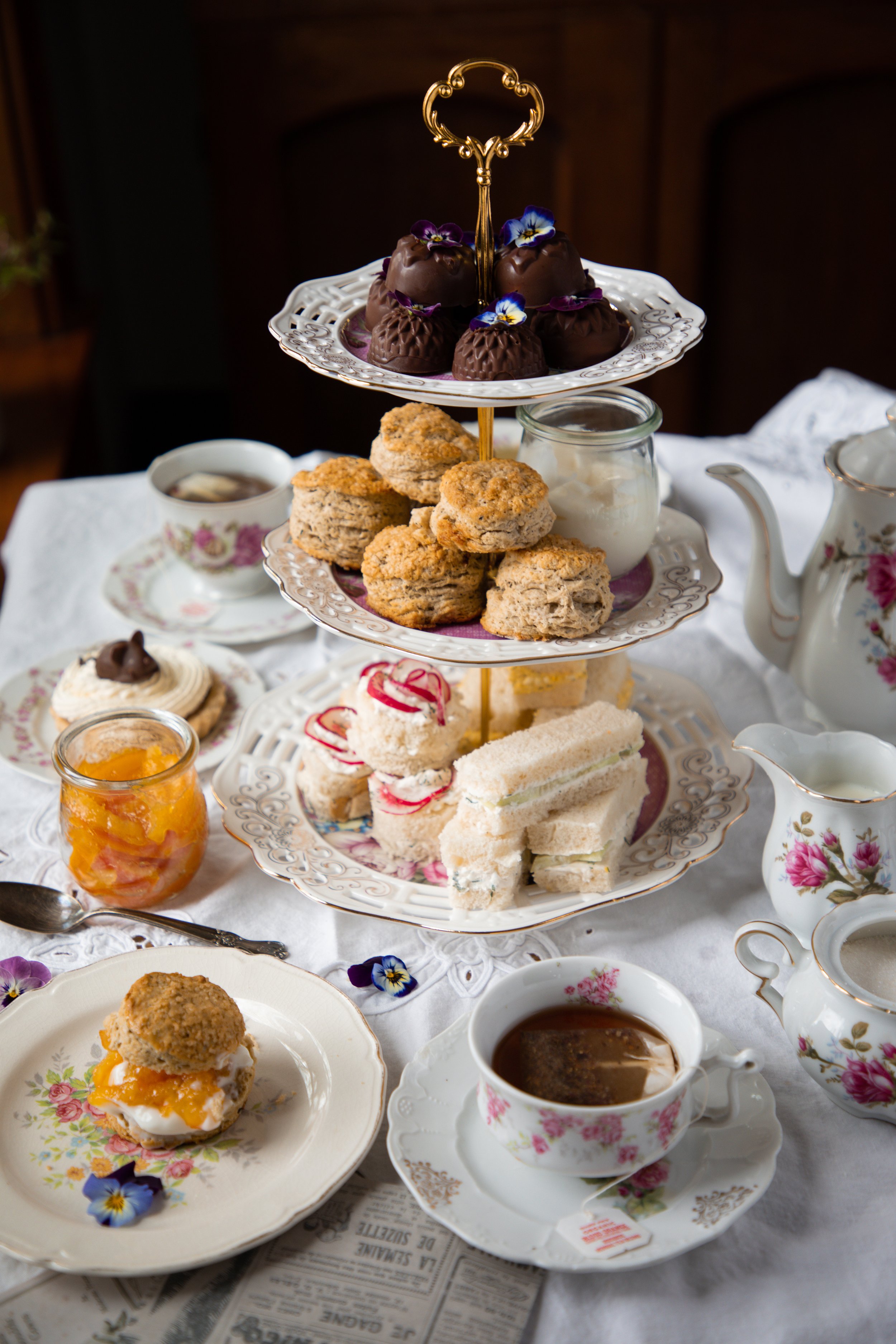This detailed photograph captures an elegant three-tiered tray garnished with an assortment of desserts, surrounded by a tea set, all arranged on a white tablecloth. The three-tiered tray, adorned with a gold handle at the top, features progressively larger porcelain plates that are trimmed in gold and display intricate designs in their centers. The topmost tier showcases decadent black chocolates, while the middle tier presents delicate cream puffs adorned with blueberries, alongside what appears to be a small cup of peaches or perhaps a white fluid. The bottom tier offers enticing strawberry shortcakes. Adjacent to the tray, neatly arranged, are several teacups filled with tea, each resting on matching saucers. A pot of water for brewing tea stands at the top center, alongside a jar that likely contains marmalade or apricot jam, accompanied by a spoon. A separate small cup bears creamer, and a silver spoon rests nearby to complete the meticulously matched tea set ensemble. Each piece—from the teapot to the cream-filled croissants—contributes to the sophisticated tea party ambiance depicted in this image.